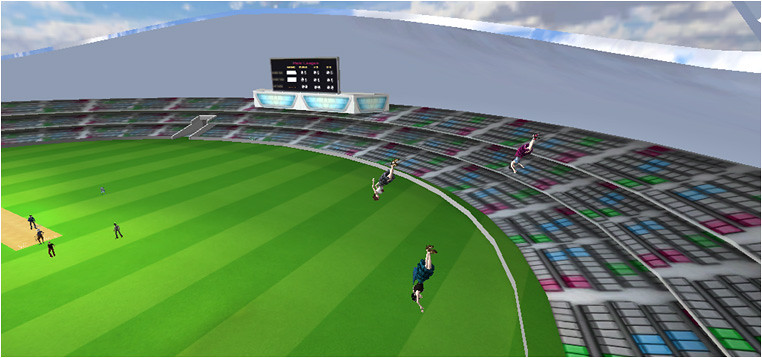This computer-generated image, likely rendered on a PC, depicts a sports field. It is unclear whether the field is intended for baseball, football, or soccer, but it features meticulously detailed green and dark green stripes that cover the majority of the surface. In the lower-left corner, there is a small square patch of dirt, adding texture to the digital terrain.

Scattered across the field are tiny avatar figures, representing players. Curiously, several avatars appear to be falling from the sky. Among these, one is dressed in a turquoise dress, while another sports purple shorts, and the attire of the other figures is indistinguishable.

Surrounding the field, there are spectator stands that span the entire perimeter of the facility, creating a rounded, enveloping structure. These stands are vividly colored in shades of gray, blue, purple, and even some green, adding an eclectic backdrop to the scene. The image is an intriguing blend of digital artistry and surreal elements, capturing a unique, otherworldly sporting event.